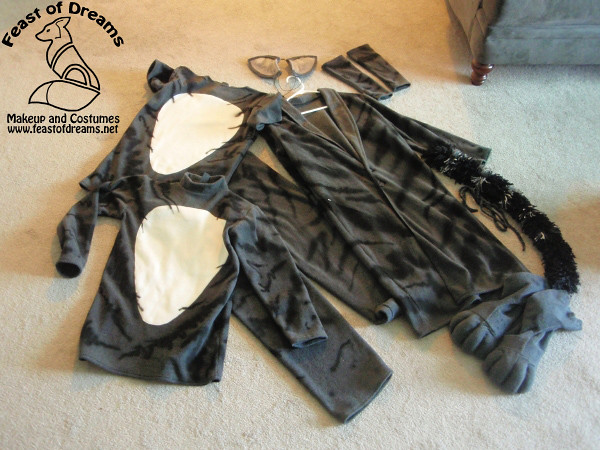This vibrant, full-color photograph captures the contents of a detailed costume laid out on a tan carpet in what appears to be a home setting. Central to the image is a blue piece of furniture with a wooden leg, adjacent to which lies the meticulously arranged costume components. The outfit is primarily grey with black stripes, designed to resemble a cat’s fur pattern. Included in the ensemble are two shirts: a short-sleeved t-shirt and a long-sleeved turtleneck, both featuring a white patch on the chest mimicking a cat's belly. Accompanying these are matching pants, a long jacket, and various accessories. Gloves designed to look like paws and a tail enhance the feline theme, and the costume is completed with a pair of cat ears. The image also showcases a logo for "Feast of Dreams" along with a fox drawing, and the website "www.feastofdreams.net" promoting makeup and costumes.